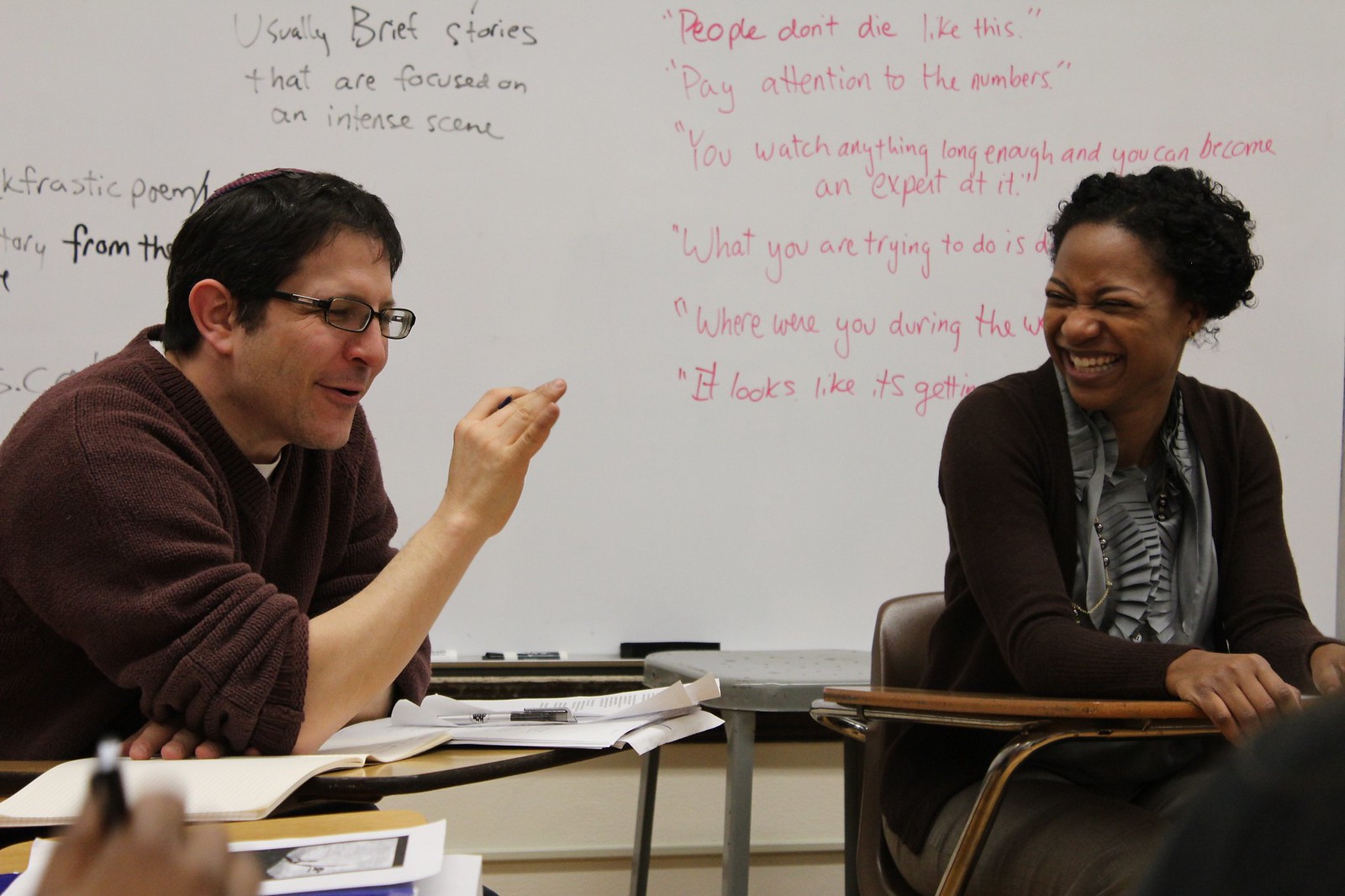The photograph depicts two individuals in what appears to be a classroom setting, seated at school desks with a whiteboard in the background adorned with a mix of black and red text. The text on the whiteboard includes a large red line at the top that reads, "people don't die like this," followed by phrases such as "pay attention to the numbers" and other less discernible lines.

Seated on the left is a middle-aged man, likely in his late 30s or 40s, with short dark hair and dark glasses. He is clean-shaven and dressed in a dark brown sweater with the right sleeve pulled up to his elbow. His right arm is bent and resting on the desk, holding papers and a pen. His expression suggests he is either explaining something or making a joke.

To the right is a dark-skinned woman with curly black hair. She is also dressed in a dark brown sweater, paired with a gray blouse featuring black horizontal stripes and a gray skirt. She sits with her hands clasped on the desk, looking at the man and smiling, seemingly amused by his words. In the backdrop, there is a grey stool near the whiteboard, which holds a duster and a marker at its bottom edge, contributing to the classroom ambiance.